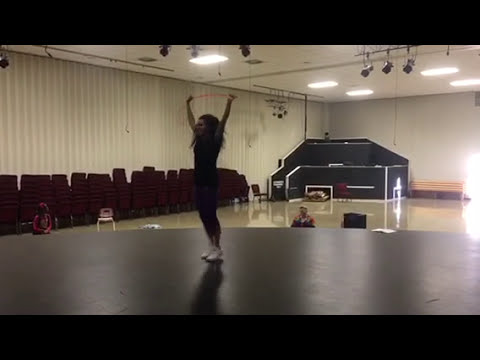The color photograph, in landscape orientation, captures a performance on a shiny black stage in an auditorium. At the center of the image is a teenage girl with fluffy hair reaching just below her shoulders, dressed in a black suit that extends below her knees, paired with white sneakers. She stands slightly to the left of the stage's center, facing right, with her arms triumphantly raised above her head, clasping a pink line or wand between her hands. The background reveals a shiny, light-yellow gym floor reminiscent of a basketball court, with several chairs: one man seated in the center, an empty chair to his right, and another empty chair farther left. Stacked chairs are visible on the left side of the scene. The wall behind the stage is a dirty white color with rippled textures, and the ceiling, also white, features recessed lights and unlit hanging lights. The overall ambiance suggests a practice session or rehearsal, with some sporting gear in the corner adding to the gym-like environment. The detailed realism of the photographic style emphasizes the scene's clarity and representational quality.